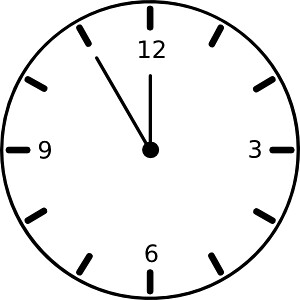This image features a simple, digitally drawn clock on a stark white background. The clock is a perfect black circle, marked by four main numbers: 12 at the top, 3 on the right, 6 at the bottom, and 9 on the left, rendered in a standard, non-bold black font, possibly Arial. The remaining hours are indicated by bold black tick marks, with no additional minute markers in between. Two straight black hands, a shorter hour hand, and a longer minute hand, indicate the time as 11:55, converging at a small black circle in the center. The overall design is minimalistic and monochromatic, emphasizing clarity and simplicity.